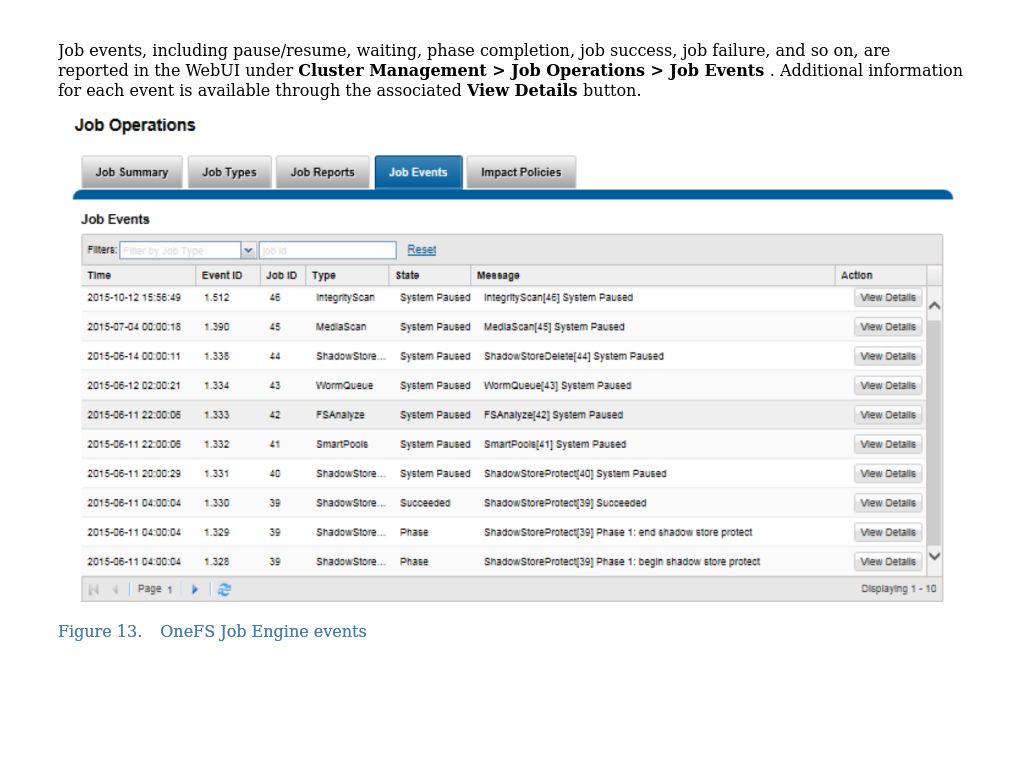This screenshot captures a detailed view of job events within a web user interface (UI) dedicated to cluster management and job operations. It displays an array of job-related activities, including options to pause and resume jobs, and reports on phase completion, job successes, job failures, and more. Each job event is accompanied by comprehensive additional information, accessible through the "View Details" button.

The interface features several tabs including "Job Summary," "Job Types," "Job Reports," "Job Events," and "Impact Policies," offering various filtering options. Users can filter events by job type, job ID, and reset filters as needed. Each event is timestamped and dated for accurate tracking. For instance, the first row indicates a job event that occurred on October 12, 2015, at 15:56, while the next row lists an event from July 4, 2015. This organized and detailed layout aims to facilitate efficient monitoring and management of job events within the cluster.